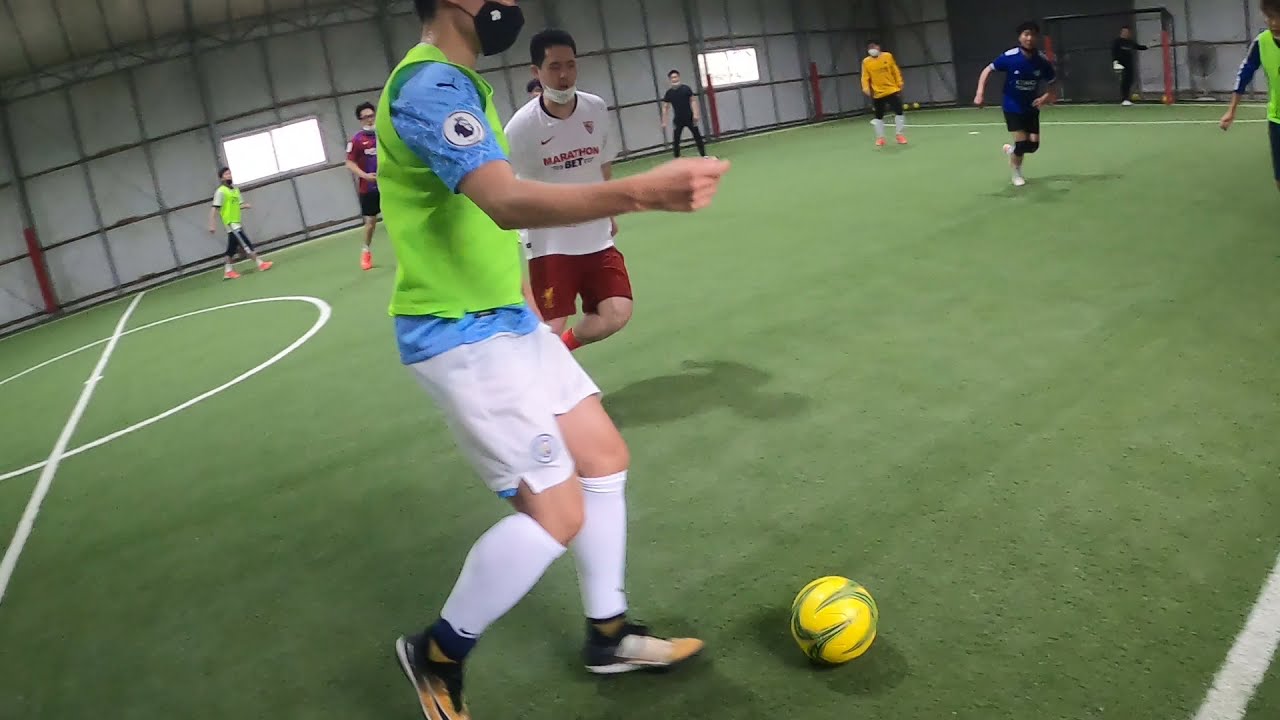The image depicts an indoor soccer game set on a green artificial turf field with white stripes. Central to the scene, a player in a bright green vest over a blue t-shirt stands poised to kick a yellow and green soccer ball. He is wearing white shorts, white socks, and colorful tennis shoes, and he has a face mask on. To his left, another player dressed in red shorts, a white and red t-shirt, and red socks is approaching. The players do not appear to be wearing standardized uniforms, with some in bright green vests, suggesting an informal match possibly with teams divided by those wearing the vests and those not. There are other players in the background, some running towards the ball while others stand further away, waiting. The setting is clearly indoors, as indicated by the surrounding walls and the light spilling through two windows in the background. The absence of referees and a scoreboard further implies this is a casual, possibly recreational game. Most of the players appear to be of Asian descent, hinting that the location could be in an Asian country.